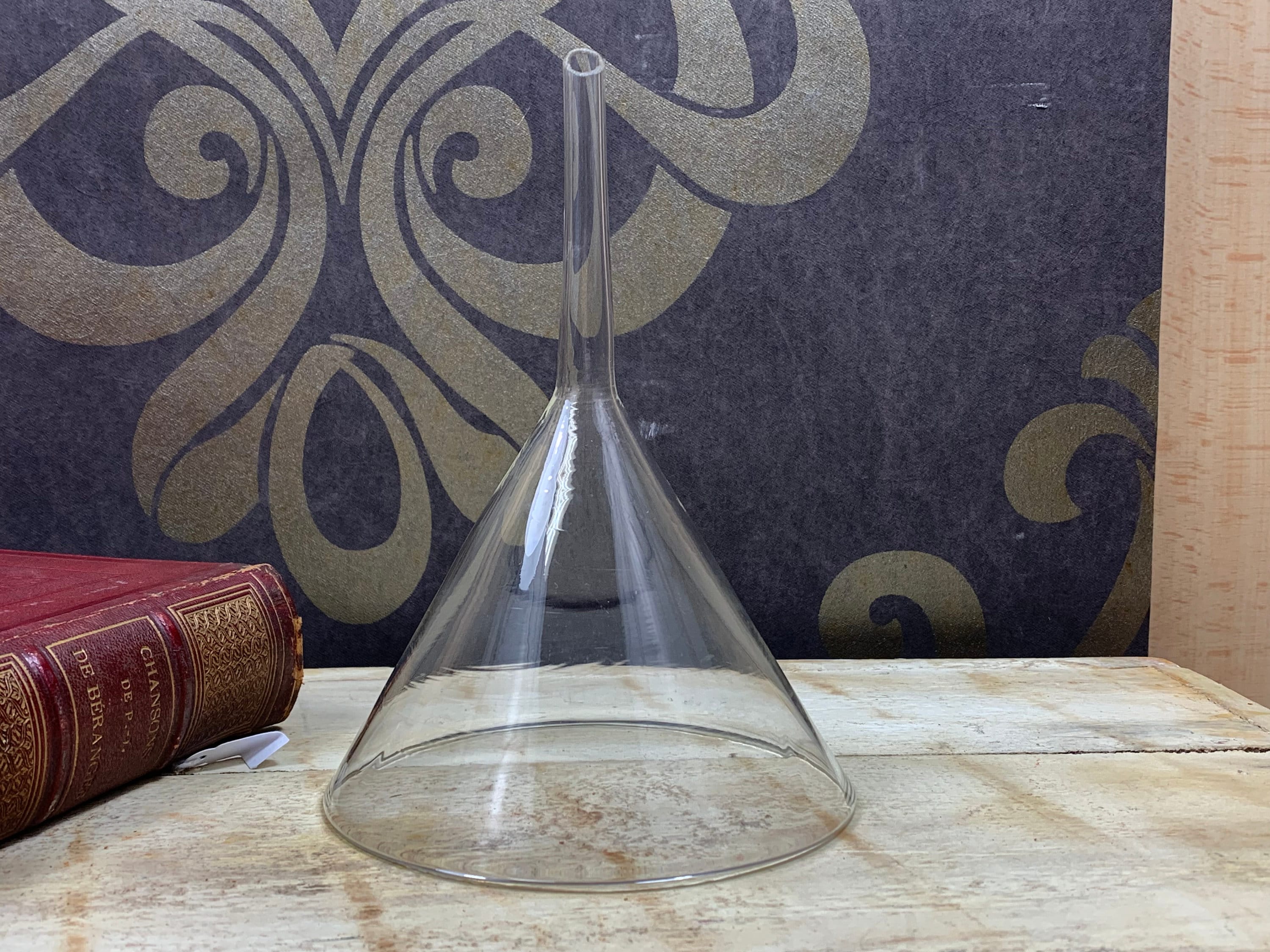The image depicts a vintage glass container with a conical body and a completely flat bottom. The container features a narrow glass tube extending from the top, reminiscent of a scientific or medical beaker. The transparent glass structure is perched on a white and beige wood surface, with visible grain lines in brown vertically crossing the tabletop, which resembles a handmade wooden end table. To the left of the container, there is a large, closed, maroon-colored leather-bound book, adorned with gold leaf designs and French writing on the spine, suggesting its vintage nature. In the background, a stylish wallpaper with a black backdrop showcases an intricate golden floral pattern, adding a regal touch to the setting.